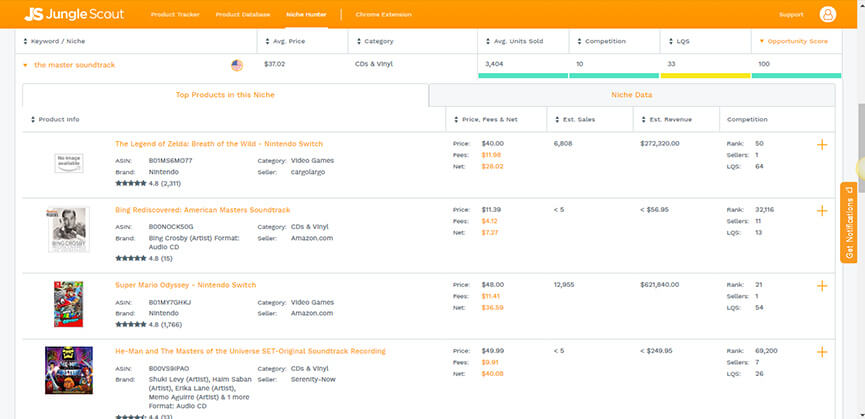A detailed screenshot showcasing the Jungle Scout interface on a white background. The screenshot features an orange header displaying the text "JS Jungle Scout." In the center, there's a prominent white circle with an orange profile icon. The interface is divided into various sections including fields labeled "Keyword," "Average Price," "Category," "Average Unit Sold," "Competition," and "Logs." One noticeable element is an opportunity score highlighted in orange.

Additional elements include product information typically listed alongside various metrics such as price, person, net, estimated sales, estimated revenue, and competition level. There is also an orange text heading for "The Legend of Zelda: Breath of the Wild - Nintendo Switch" with details like "Price: $40," "Fees: $11," and "Net: $26." The American flag icon is also visible, situating the product information within the US market context. The text in some sections appears small and might be challenging to read.